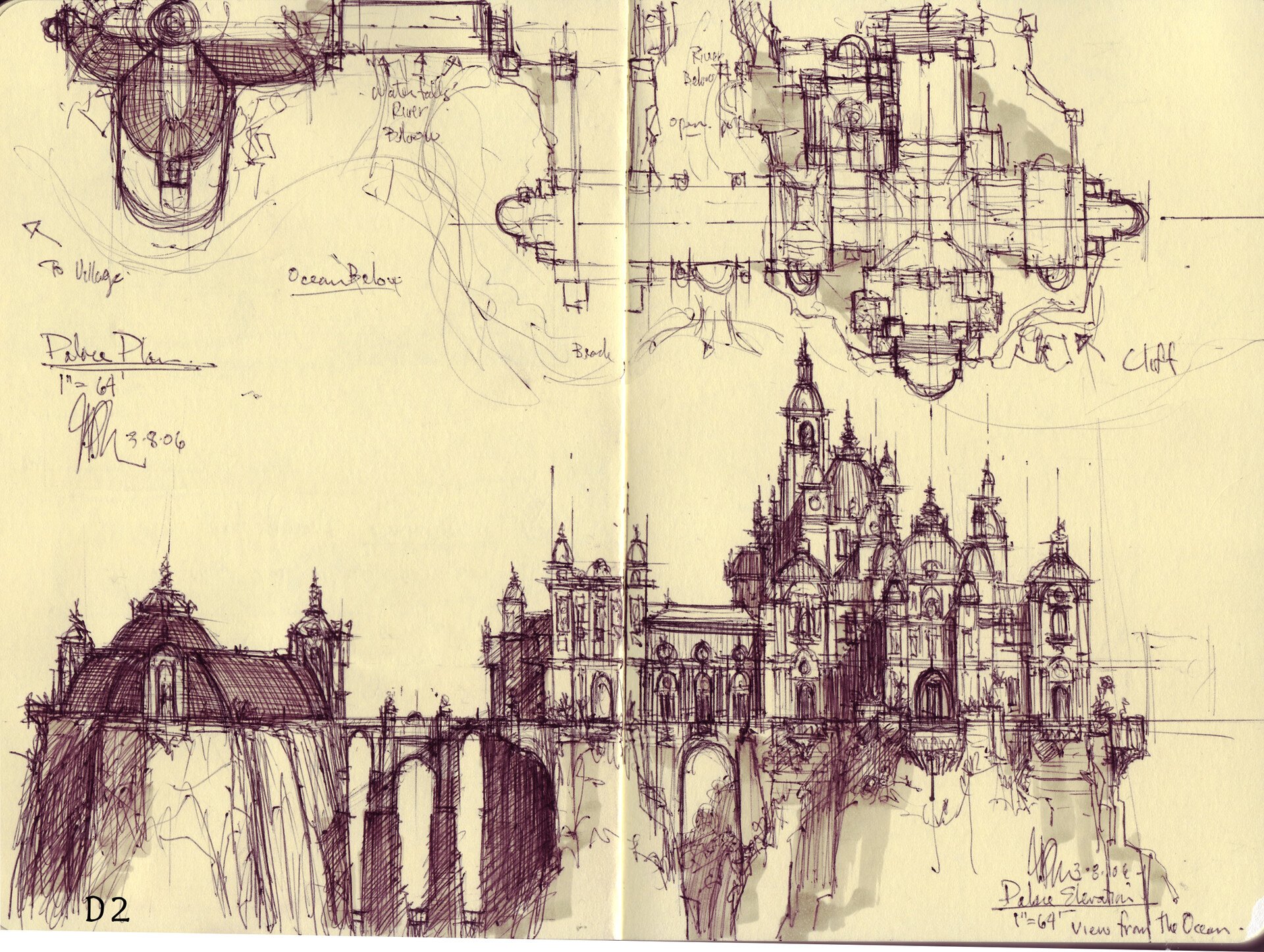The image depicts a highly detailed sketch on a cream-colored, flat sheet of paper, likely taken from a sketchbook, with the seam visible down the center. The intricate sketch appears to feature a large, elaborate palace or castle situated atop a mountain or cliff, complete with multiple gothic-style towers and pointed tops. The lower half of the sketch comprises a side view of this grand structure, highlighting its position next to water with possible reflections, waterfalls, and a river below. This part of the drawing includes details such as a pillared bridge on the left and various direction arrows indicating elements like the ocean, village, and cliff. On the upper half of the image, there's a top-down view showcasing the geometric floor plans and layout of the buildings. The page carries a signature and date in the bottom right, alongside labels and annotations like "palace elevation" and "one inch equals 64". The paper appears to be either yellowed or naturally cream, suggesting age or intentional coloration. The sketch serves as an elaborate, Gothic-style architectural proposal or concept sketch, expertly rendered in black ink or pencil.